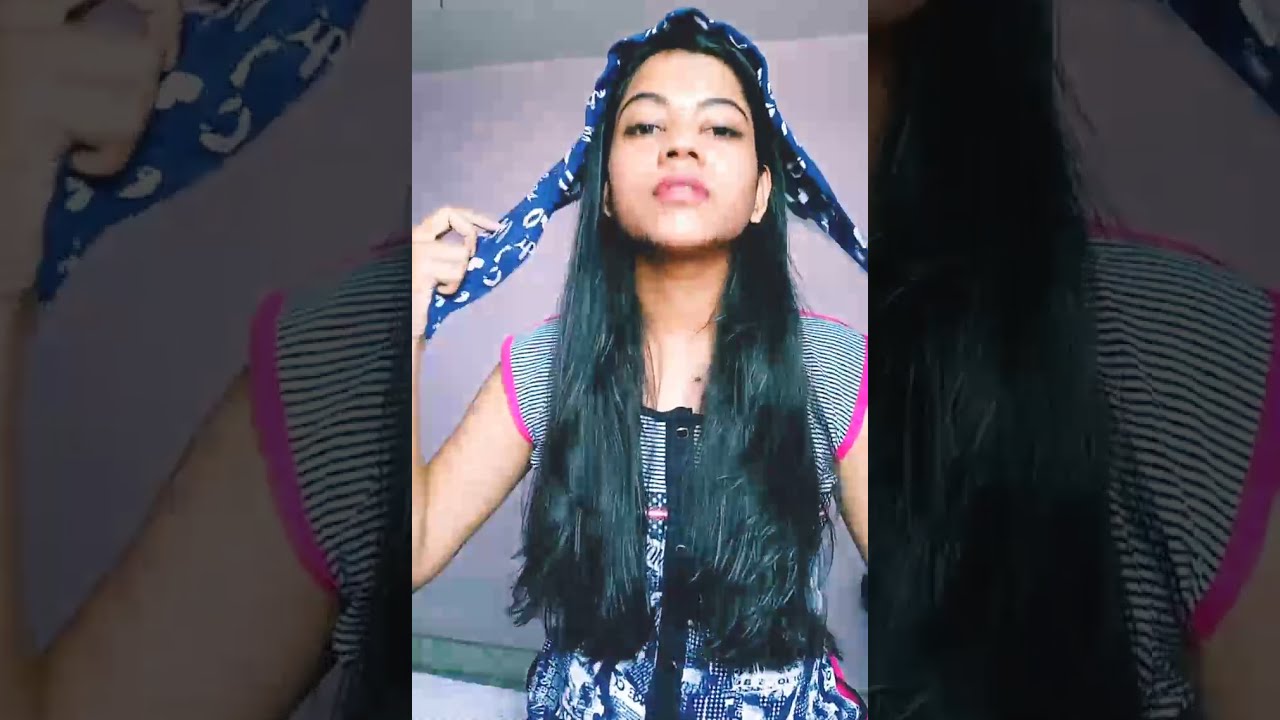The image features a young woman with long black hair flowing down to her waist, some of which is draped over her shoulders. In the center of a three-panel, rectangular layout, the brightly lit middle panel highlights her as she looks directly at the viewer. Her mouth is slightly open, revealing a contemplative expression. She is tying or adjusting a blue kerchief or scarf around her head, its tails falling on either side of her face. The scarf has intricate designs, adding a touch of intricacy to her otherwise straightforward attire.

Her attire consists of a short-sleeved smock-type shirt. The shirt features black and white stripes along the shoulders, transitioning into blue and white designs below, accented with pink trimming around the sleeves and down the sides. Additionally, there is a vertical black stripe with buttons running down the front of the shirt.

In the background, there is a predominantly gray wall with a hint of a gray ceiling, bordered by a pinkish-purple section below and a green bottom border, giving the setting an unfinished, raw look reminiscent of concrete. To the right and left of the central panel, dimmed close-up versions of the middle image provide additional context, emphasizing the woman’s face and attire while maintaining a focus on her thoughtful expression.